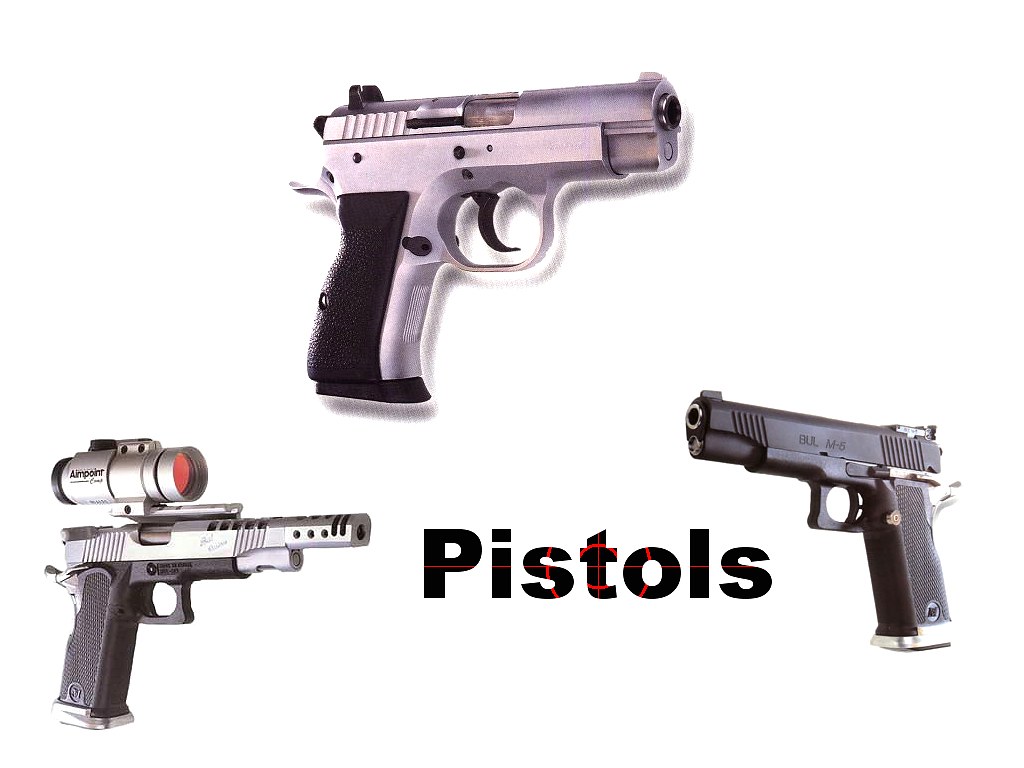The image features three distinct handguns arranged around the prominent black text "Pistols." The text incorporates parts of a red target embedded among the letters "ST" and "O." At the top, there is a compact revolver with a silver body, black handle, and black trigger, pointing to the right. Moving clockwise, to the left, there's a mostly black handgun with a touch of silver trim, adding a sleek look to its design. On the right side, there is a more tactical-looking pistol equipped with a scope, resembling the features of a lightweight, square-design Glock. All three pistols appear to be made of metal and could be interpreted as either real firearms or novelty items.